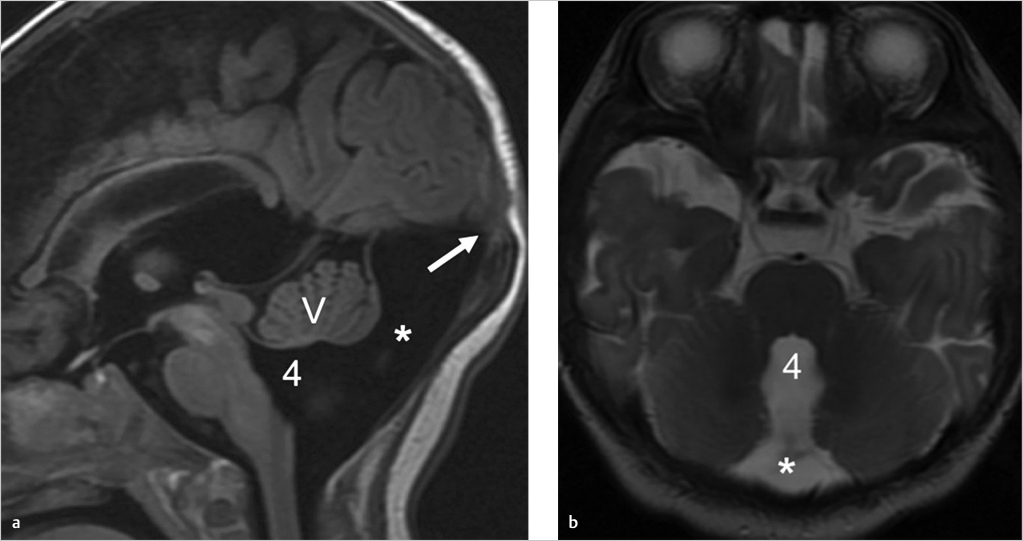The image displays two professional black and white x-ray or scan photos of a person's head, highlighting the brain. The first image, labeled 'A', presents a side profile of the skull revealing the brain matter within. This image includes annotations such as a 'V', the number '4', an asterisk, and an arrow pointing to the back of the head. The second image, labeled 'B', offers an overhead, top perspective of the skull, similarly allowing visibility of the brain. This image also features the number '4' and an asterisk near the back of the head. Both images, devoid of any additional texts or labels, are positioned side-by-side and offer a detailed look at the scanned brain matter, giving an impression akin to x-ray cross-sections.